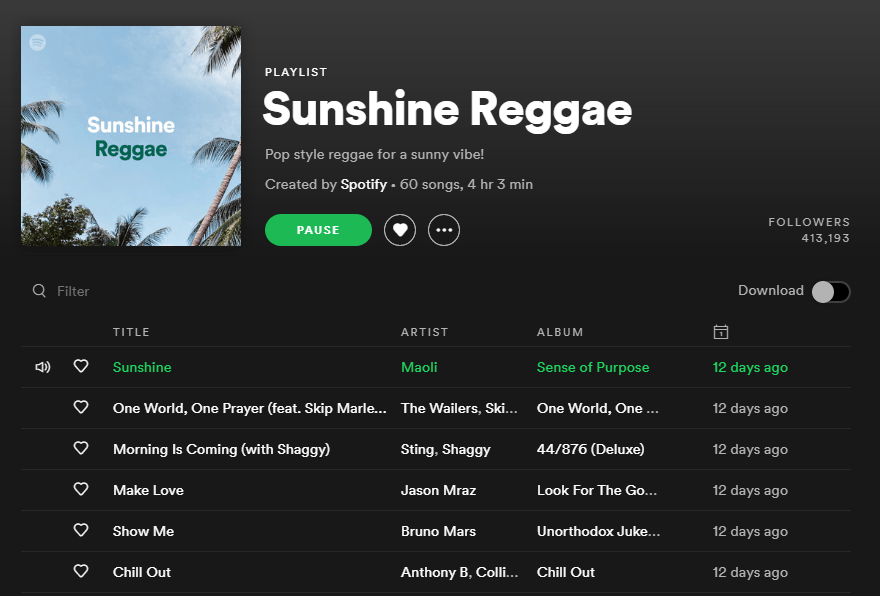This is a screenshot of a page from a music streaming app, likely Spotify. The upper half of the page serves as a detailed header for a playlist titled "Sunshine Reggae." On the left-hand side, there's a small image featuring a serene backdrop of a setting sun with the tips of palm trees silhouette along the border. The word "Sunshine" is prominently displayed in white, with the word "Reggae" in green just below it, creating a cheerful, tropical ambiance. To the right of the image, in smaller white letters, it says "Playlist."

In bold, white lettering, the title "Sunshine Reggae" is reiterated below the image. Beneath the title, a brief description reads: "Pop style reggae for a sunny vibe," encapsulating the playlist's mood. Further down, it mentions the playlist was "Created by Spotify" and contains "60 songs, 4 hours, 3 minutes" of music.

Below this information, there are three interactive icons: a green radio dial labeled "Pause" in white text, a circle with a heart icon for marking favorites, and a circle with three dots for additional options.

The lower portion of the page is organized into four columns titled "Title," "Artist," "Album," and "Date Added," listing a series of songs included in the playlist.